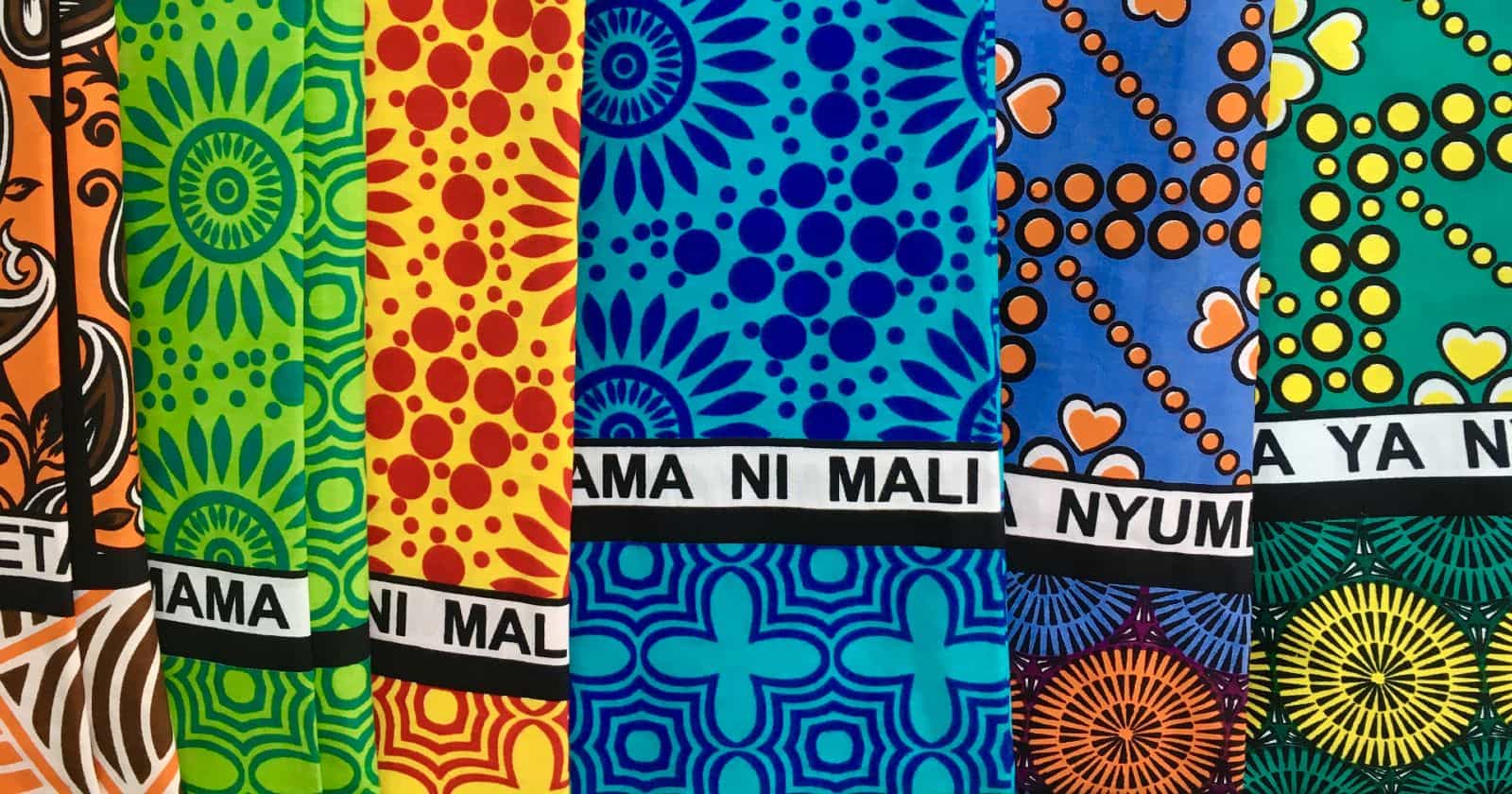The image depicts an array of six colorful scarves, each detailed with intricate designs and the phrase "Mama Nimale" prominently displayed. From left to right, the first scarf is vibrant orange adorned with intricate white and black patterns, and features the letters "E-T-A" on a white background. Next is a green scarf, decorated with darker green sun motifs and the word "Mama" in black on a white stripe. The third scarf showcases a bright array of red polka dots on a yellow background, with the letters "N-I-M-A-L" in black against a white backdrop, interspersed with floral elements. Following this is a blue scarf with darker blue polka dots and sun-like designs, displaying the letters "A-M-A-N-I-M-A-L-I" alongside blue plus symbols and smaller polka dots. The fifth scarf combines a blue background with orange hearts and polka dots, featuring the letters "N-Y-U-M", and below, there are pinwheels in various colors including orange, purple, and blue. The final scarf returns to a green color, embellished with yellow hearts and polka dots, the word "A-Y-A-N" in black text on a white background, and a bottom border filled with green and yellow pinwheels. Displayed in a linear arrangement, these scarves not only showcase a rich palette of colors—orange, green, yellow, and blue—but also an array of patterns, including polka dots, suns, pinwheels, and hearts, making for a visually engaging and detailed composition.